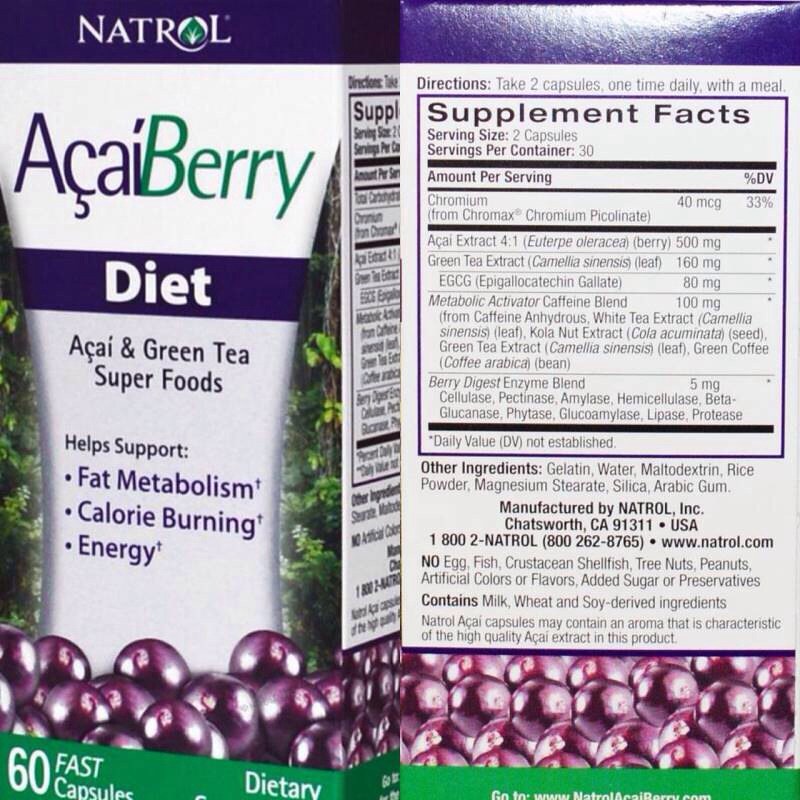The image features a high-quality photograph of a product box for Natrol Acai Berry Diet, designed as an advertisement, likely for a website. The product packaging is showcased in two side-by-side images: the front of the box on the left and the back on the right. 

The front of the box sports a clean, white background with the brand name "Natrol" in white text, with a distinctive green leaf inside the letter "O." Below this, the words "acai" in blue and "berry" in green are prominently displayed. Beneath them is a purple stripe containing the word "diet" in white text. A detailed description follows, stating, "Acai and green tea superfoods help support fat metabolism, calorie burning, and energy," printed on a lavender background. The bottom section of the front displays an image of purple berries set against a leafy nature background, ending with a green stripe that reads "60 fast capsules, dietary supplement."

The right side of the image shows the back of the box, which includes the Supplement Facts label providing nutritional information. It suggests taking two capsules once daily with a meal and lists the ingredients. The back design is consistent with the front, featuring grape imagery and the same nature-themed background motifs.